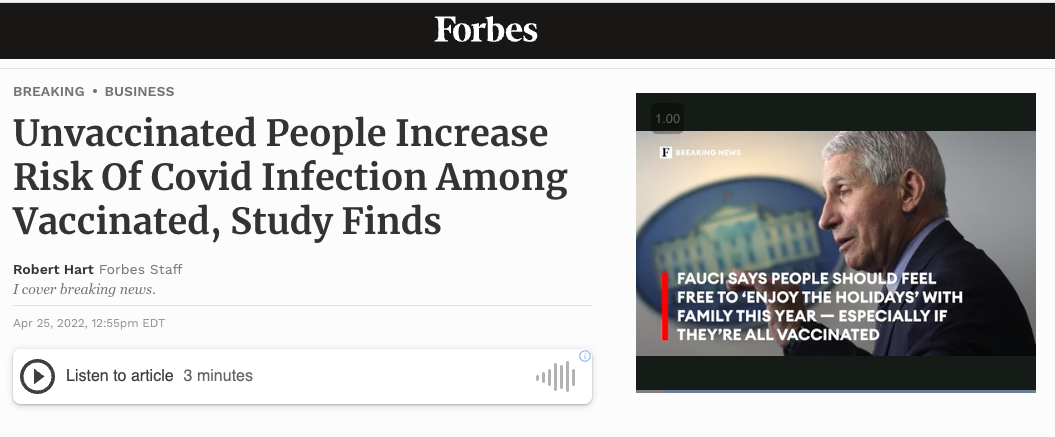This is a horizontal image captured from a computer or smartphone device, showcasing a news article from Forbes. At the top of the image, there is a black, long, thin, rectangular strip displaying the Forbes logo in white. Below the strip, "Breaking" and "Business" are written in gray text.

The main headline of the article is prominently displayed in bold text and reads: "Unvaccinated People Increase Risk of COVID Infection Among Vaccinated, Study Finds." Beneath the headline, "Robert Hart" appears in bold, smaller text, followed by "Forbes Staff" in gray. The author's brief description reads, "I Cover Breaking News," followed by a thin, gray line.

The date and time of publication are listed below the line: "April 25, 2022, 12:55 EDT." Additionally, there is a small box with an icon featuring a circle and triangle, indicating an audio option to listen to the article, labeled "Listen to article 3 minutes" with visualization of sound waves.

On the left side of the image, there is a photograph of Dr. Anthony Fauci with a red vertical line. In white text, the photo caption states: "Fauci says people should feel free to enjoy the holidays with family this year, especially if they're all vaccinated."